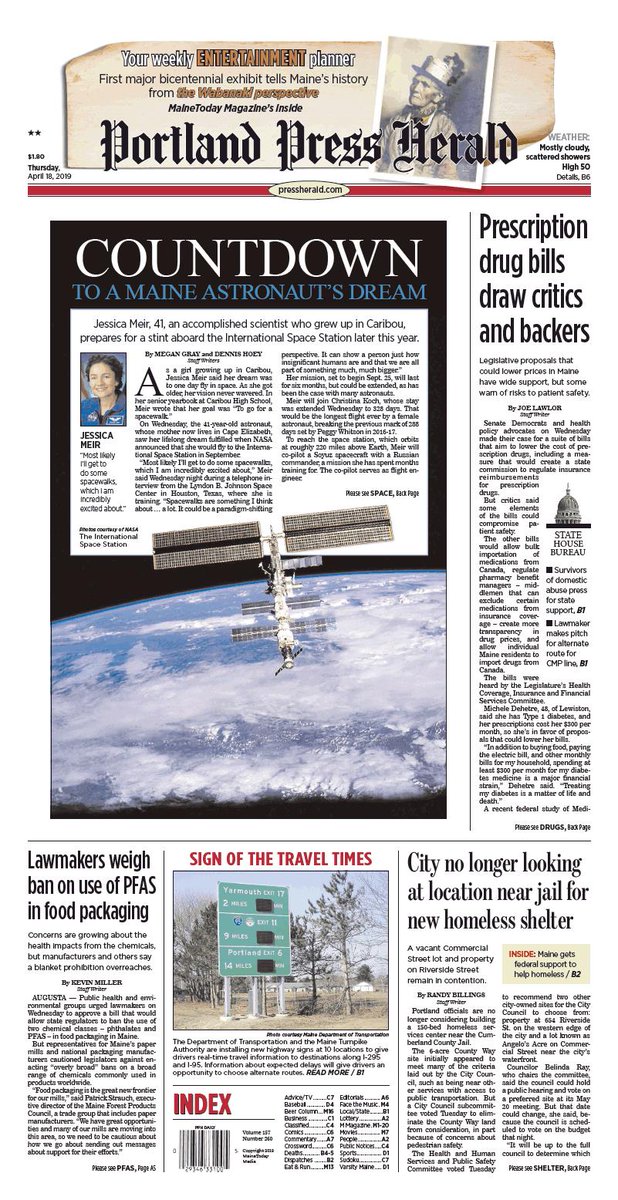This image shows the front page of the Portland Press Herald, dated Thursday, April 18, 2019. The layout features several articles, many accompanied by pictures. At the top, a banner announces "Your Weekly Entertainment Planner," highlighting the main feature, "First Major Bicentennial Exhibit Tells Maine's History from the Wabanaki Perspective." It also mentions that the "Maine Today" magazine is included inside.

Prominently displayed in the center is the headline "Countdown to a Maine Astronaut's Dream," focusing on Jessica Meir, a 41-year-old accomplished scientist from Caribou. The article details her preparations for an upcoming mission aboard the International Space Station later that year. Featured within the segment is an inspirational quote from Meir: "Most likely I'll get to do some spacewalks, which I am notably excited about." Accompanying the text is a striking image of the International Space Station orbiting above Earth, emphasizing the grandeur of her upcoming journey.

Additional articles and photographs fill the page, providing a varied and engaging snapshot of the day's news and noteworthy stories.